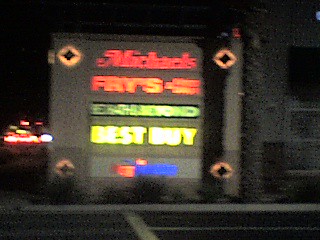The image depicts a nighttime scene, evidenced by the dark sky occupying the upper left portion of the frame. Dominating the view are the illuminated signs reminiscent of those found in an outdoor shopping center or mall. Although slightly blurred, the neon lights shine vividly. At the top of the signage array, the name "Michaels" is prominently displayed. Below it, an orange-colored "Fry's" sign follows. Next, a "Bed Bath & Beyond" sign appears, either in yellow and black or white and black. Further down, a yellow sign for "Best Buy" becomes visible before the image starts to lose clarity. At the bottom, a red and blue rectangle hints at an unidentifiable store name due to the heavy blur. Along the side of the image, a store is marked by a large red and blue rectangular sign, though its specific identity remains obscured.